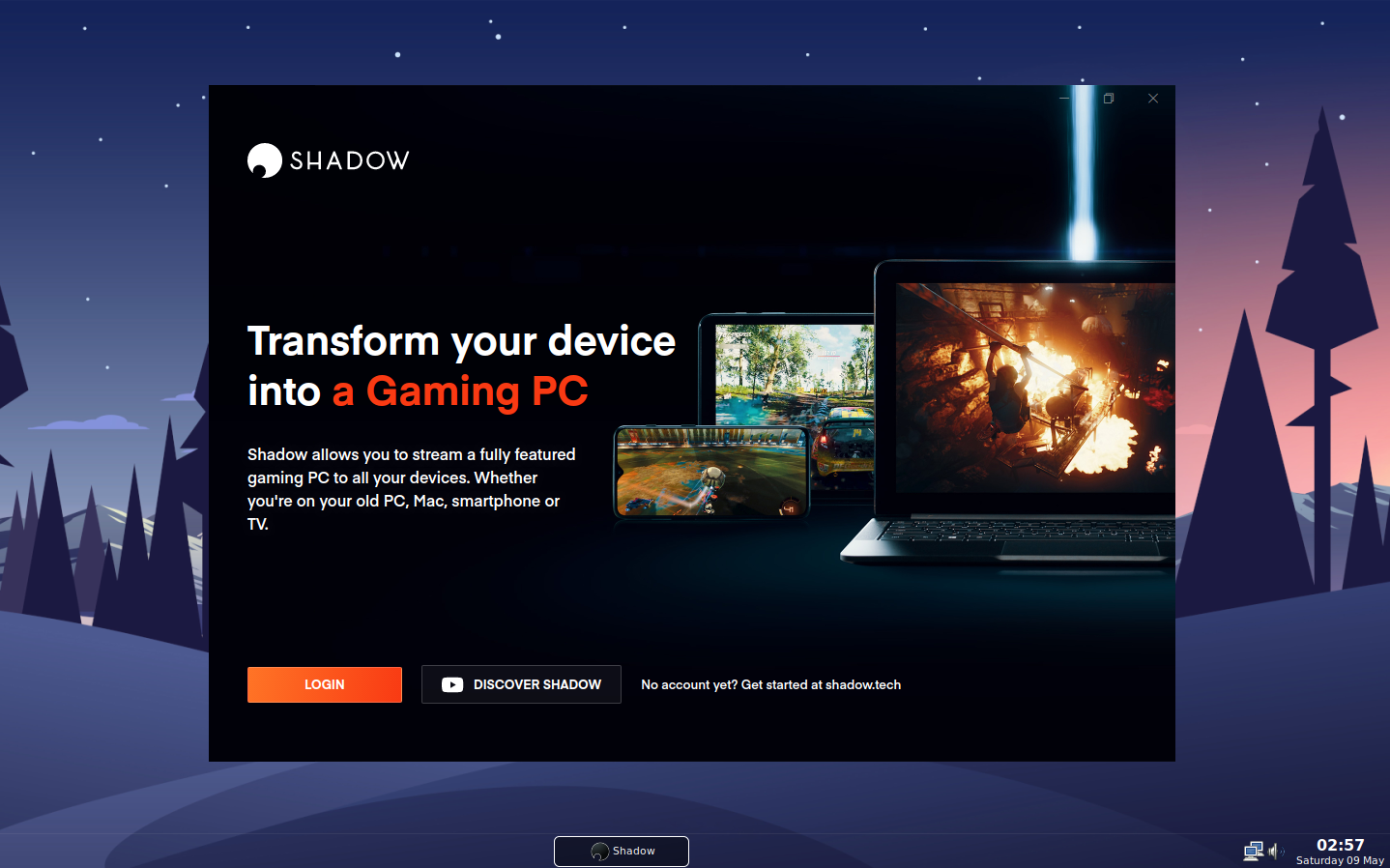A screenshot from a gaming PC advertisement, showcasing a sleek and futuristic digital rendering. In the background, an abstract landscape with sharp, light and dark blue trees is displayed against a gradient sky transitioning from deep blue at the top to a lighter blue towards the horizon. The ground reflects a similar gradient, blending blue and gray hues.

Dominating the center of the image are three horizontally oriented devices—a laptop, a tablet, and a cellphone—all set against a solid black backdrop. In the upper left corner, the Shadow icon and brand name are prominently displayed. Below the brand name, the slogan "Transform your device into a gaming PC" is split into two colors: white for "Transform your device" and vibrant orange for "a gaming PC". 

Further information is provided in a white font, stating, "Shadow allows you to stream a fully featured gaming PC to all your devices. Whether you're on your old PC, Mac, smartphone, or TV." Beneath this, an orange rectangle features the word "Log In" in white, next to a gray rectangle with the words "Discover Shadow," also in white.

To the right, additional information reads, "No account yet? Get started at shadow.tech." Below this text, a small gray rectangle outlined in white displays the word "Shadow" with the Shadow icon centered in white.

The only other text present is the time, shown in the lower right-hand corner, reading "2:57," along with the date "Saturday, 9 May."